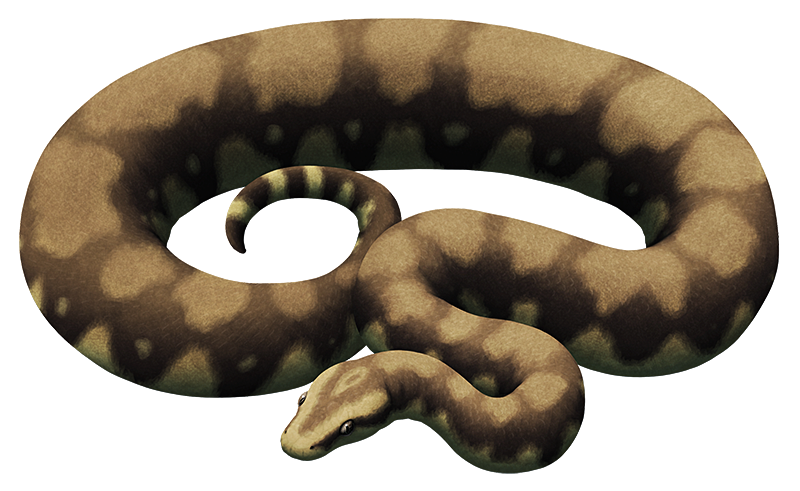This image depicts a computer-generated illustration of a snake, characterized by a lifelike yet artificial appearance. The snake, coiled into an S-shape and facing slightly left, lies calmly on a plain white background. Its coloration predominantly consists of rich, dark brown hues interspersed with lighter brown and yellowish spots that form a striking pattern. The snake's body features a series of large, light brown patches, resembling diamonds, each adorned with a small white dot at the center. This pattern continues along the snake, with the tail exhibiting a striped appearance from smaller patches. The head of the snake displays a distinctive V-shaped marking, leading down to the tip of its nose, complemented by an interesting pattern of lighter ovals and dark specks. Despite lacking scale detail, the snake's smoothly blended colors give it an airbrushed, velvety texture, making it appear more like a meticulously crafted piece of art or a model rather than a real reptile. The overall impression is of a serene, sizable snake that could be mistaken for a constrictor.